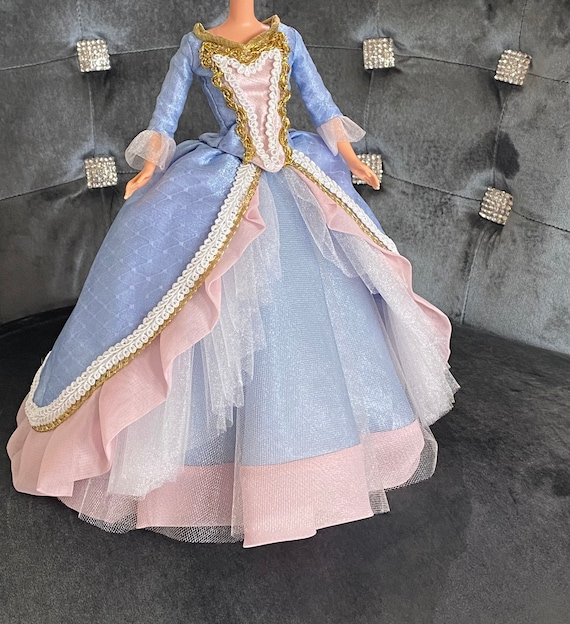This image depicts a highly detailed portrayal of a Barbie doll adorned in an opulent, upper-class Elizabethan-style dress. The doll stands against a backdrop of grayish-black velvet material that is adorned with square diamond patterns, enhancing the regal aesthetic of the scene. The focus of the image is the elaborate dress, which extends from the doll's neck downwards, accentuating the intricate design and luxurious fabric.

The dress itself is a masterpiece of craftsmanship with a predominantly bluish color scheme complemented by layers of white lace and pink ruffles. The skirt is voluminous, evoking the grandeur of Cinderella's attire, with white lace trim interspersed with ruffled layers of pink and scalloped edges. The lower part of the dress reveals an underskirt, adding to its dimension and texture.

The bodice features long blue sleeves embellished with white lace at the wrists, and a gold-trimmed neckline that delicately frames the chest area. The central panel of the bodice is adorned with a pink section that resembles a harp, potentially inscribed with text that is not discernible. This intricate detailing contributes to the overall elegance of the ensemble.

The floor beneath the doll appears to be black velvet, further enhancing the luxurious setting. The composition suggests a sense of timeless elegance and high societal status, reminiscent of aristocratic European fashion from the 1700s and 1800s. The dress’s complexity and ornate design draw the viewer's attention, making it the focal point of this captivating image.